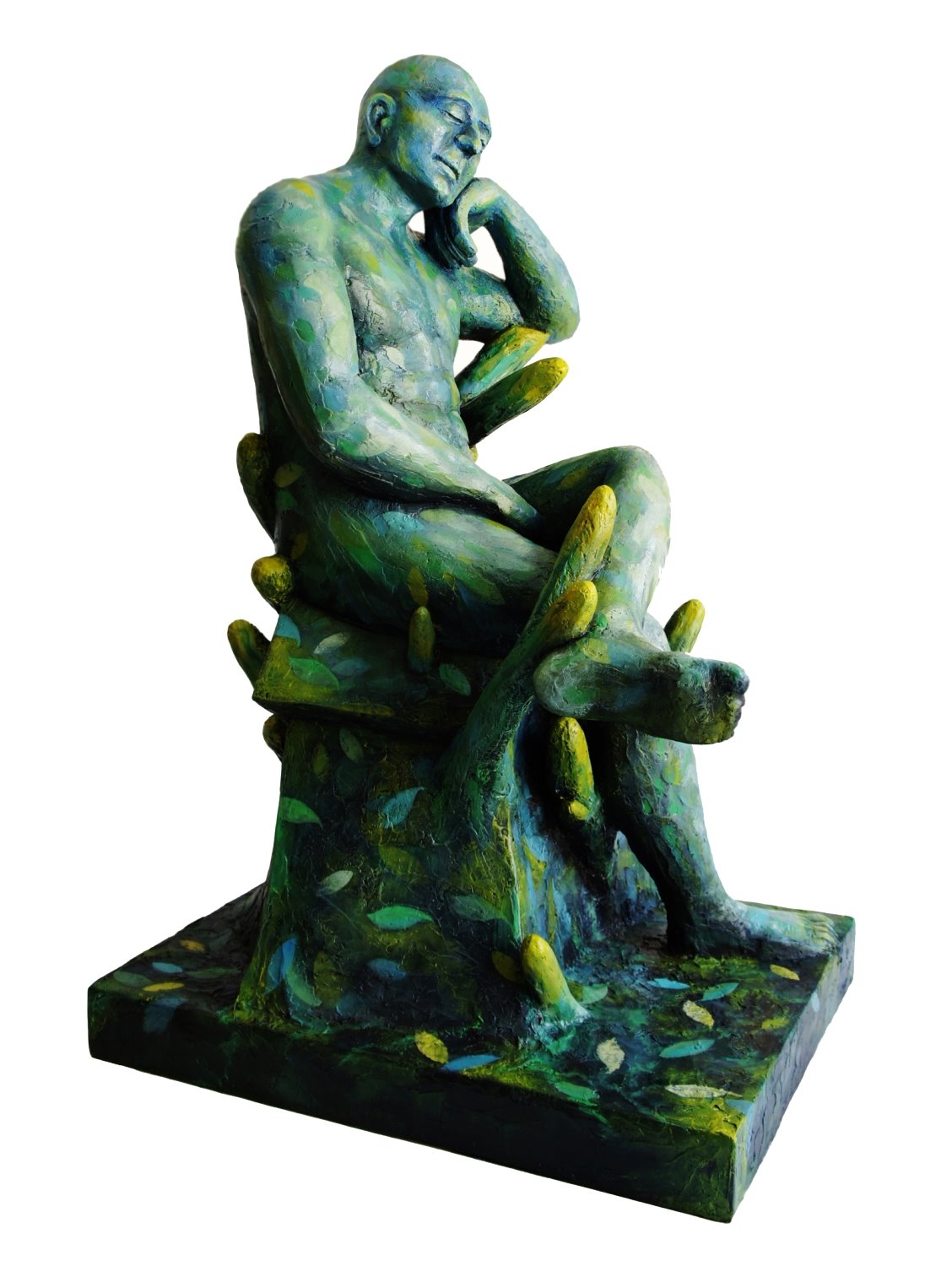The image depicts a detailed sculpture of a nude man sitting on a tree stump, which is intricately designed with various organic elements. The man, bald and well-built, leans back with one leg crossed over the other, his foot resting on his knee. His pose is contemplative, with his head slightly tilted and eyes closed, supported by one hand beneath his chin. The other hand rests across his thigh. The sculpture is predominantly green, with splotches of blue and yellow, creating a multi-color shimmer effect. The tree stump and surrounding base are adorned with leaf patterns of multiple shades of green, yellow, and hints of blue, giving the impression of a forest floor. The intricate details of the leaves and the serene expression on the man's face evoke a peaceful, daydream-like atmosphere.